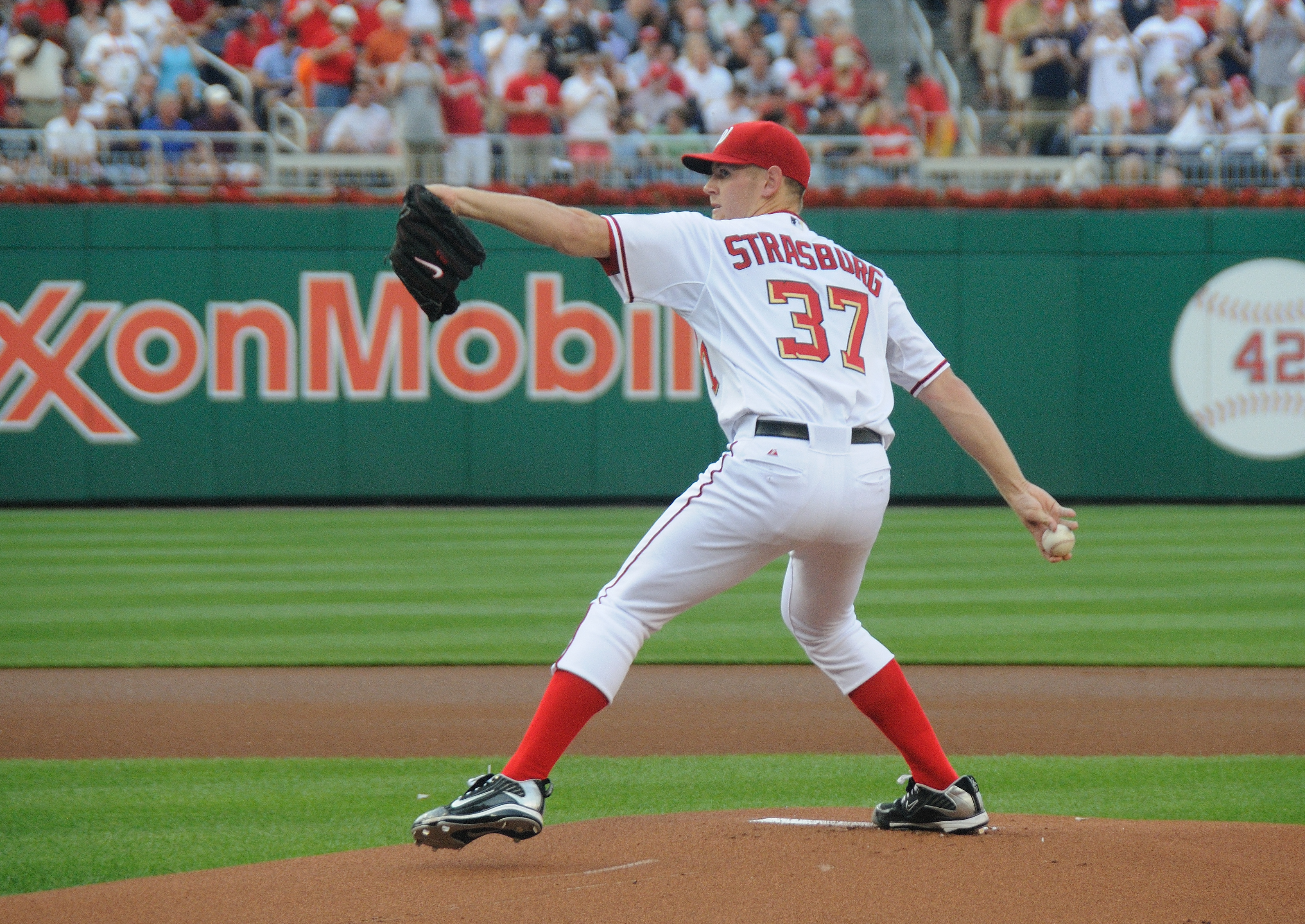The image depicts a baseball player on a pitcher's mound during a game. The player is a white male dressed in a white uniform with red accents, including red stripes down the sides of his pants and red rings around the short sleeves. On his back, in all capital red letters, is the name "STRASBURG" along with the number 37. He wears a red baseball cap and long red socks, with black Nike cleats visible on his feet. His black belt contrasts with the white uniform. The player stands with his back to the camera, holding a baseball in his right hand and a black glove with a Nike swoosh in his left. The scene includes a dirt pitcher's mound with grass visible behind him. In the background, a green wall displays an "Exxon Mobil" sign, partially obscured by the player, along with a banner featuring a baseball and the number 42. The blurred crowd in the background appears to be wearing either red or white tops.